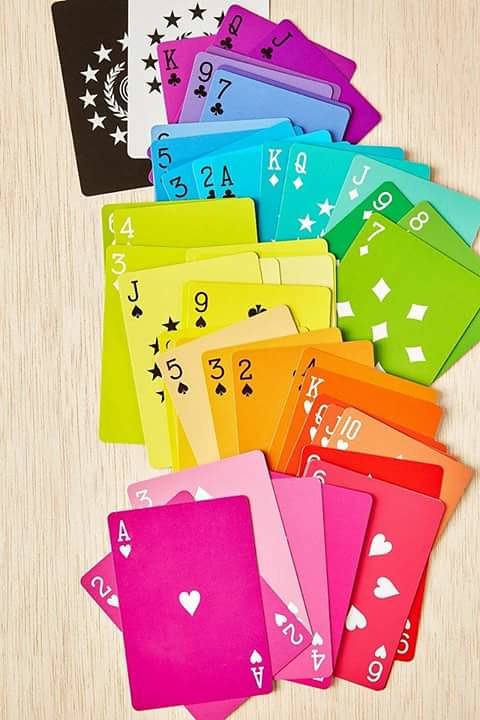This image showcases a stunning and visually captivating set of playing cards, arranged in a gradient rainbow of colors. Starting with the ace of hearts at the bottom, the cards transition from a vibrant hot pink, through a softly faded pink on the three of hearts, to a rich red by the nine of hearts. The ten of hearts begins an orange hue that continues through the face cards. This color gradually blends into yellow across the ace, two, and three of hearts, with the brightest yellow seen on the nine of spades.

Next, the jack of spades introduces a subtle washout effect, leading to a transition from lime green on the three and four of diamonds. The green progressively deepens through the seven and eight of diamonds, cultivating a richer emerald tone by the nine of diamonds. The face cards of diamonds shine with an aqua blue.

The clubs suit starts with a bright blue on the ace, two, and three, which intensifies into a deeper blue and then shifts to violet by the seven. The nine of clubs showcases a lush purple, and the club face cards culminate in a deep indigo. Additionally, the set includes two unique cards: one black and one white, both adorned with stars, adding a touch of celestial charm to this captivating collection.